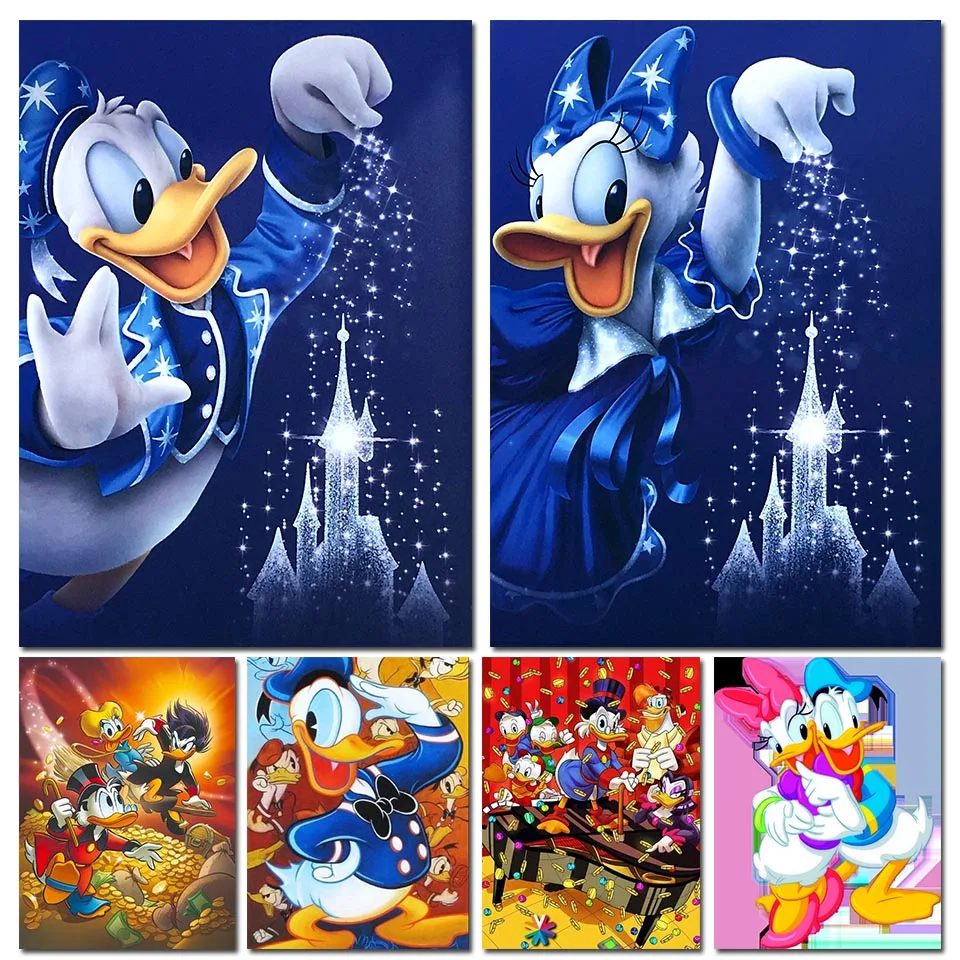The image is a detailed compilation of six Disney-themed segments. In the top row, there are two larger rectangular images, each depicting Donald Duck and Daisy Duck, respectively. Donald is wearing a vibrant, star-studded blue sailor suit, complemented by white gloves and a sailor hat with a ribbon. He is sprinkling a sparkling, star-like pixie dust onto a white silhouette of Cinderella's castle, against a dark blue background. To his right, Daisy Duck mirrors Donald's pose. She dons a blue satin dress and a large bow on her head, also sprinkling pixie dust on the castle. Both images share the same background and theme, emphasizing their magical act.

Below these two primary images are four smaller ones. The first small image shows Scrooge McDuck and characters from his series running across a vast pile of golden coins. The second image features Donald Duck saluting while wearing his classic sailor suit, set against a backdrop containing various other images of himself. The third image, once again starring Scrooge McDuck, shows him and his nephews atop a piano surrounded by falling golden coins. The final image in the bottom right portrays a heartwarming scene of Donald and Daisy Duck hugging each other; Donald is in his blue sailor outfit, and Daisy wears a pink bow. Each segment captures beloved Disney characters in charming, lively scenes, unified by a magical, fairytale ambiance.